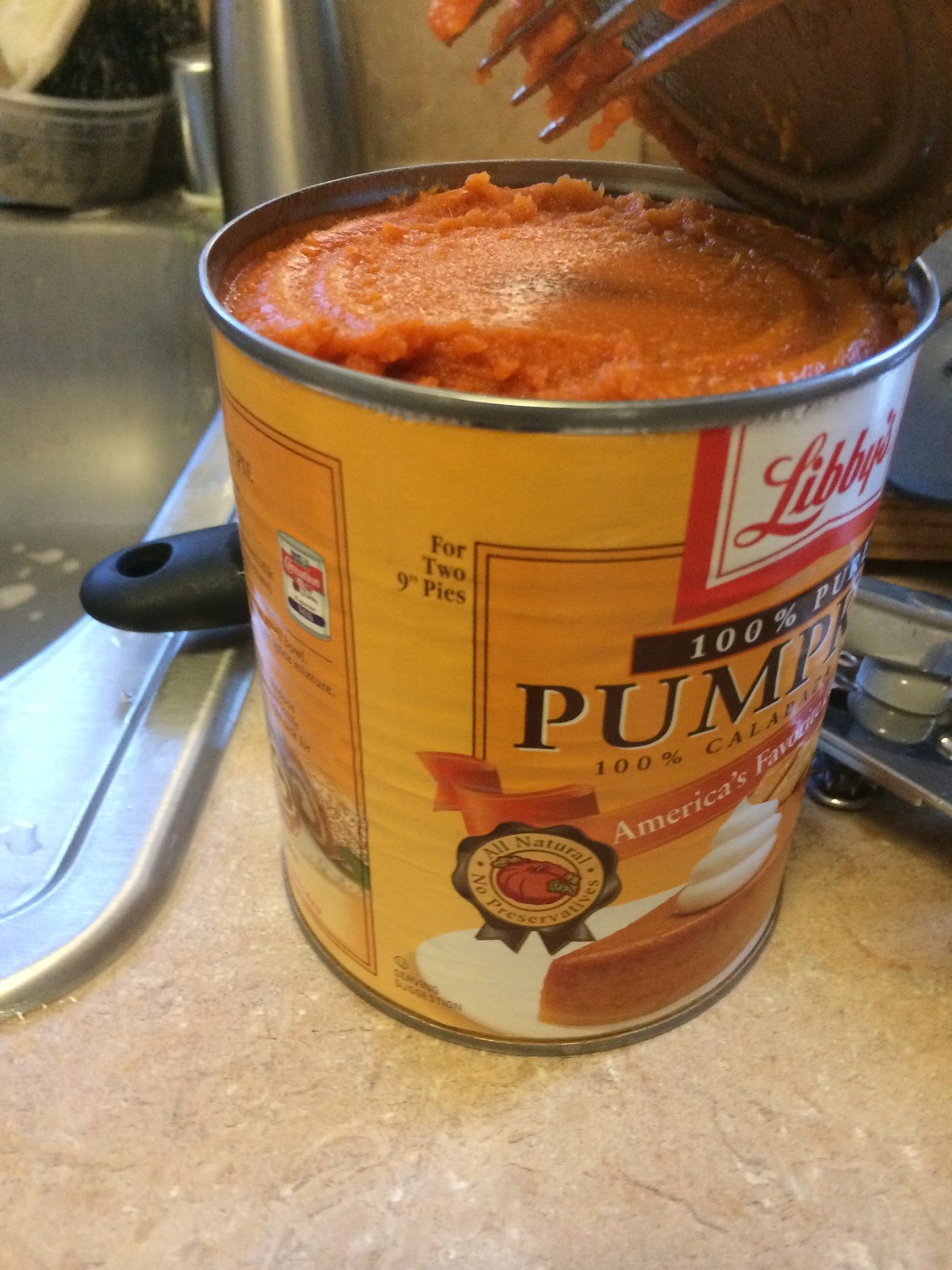This color photograph features a medium brown stone countertop as the setting. Prominently displayed on the countertop is an opened can of Libby's Pumpkin, America's favorite pumpkin brand. The label on the can is distinctive, with "Libby's" written in red and white, while the pumpkin illustration and text are in orange. A partially attached lid reveals the can’s contents—vibrant orange pumpkin puree. Resting on the edge of the can is a fork, dipped into the pumpkin, showcasing a small amount of the puree on its tines. At the bottom of the label is an image of a slice of pumpkin pie adorned with a dollop of whipped cream, and a note indicating that the can's contents are sufficient for two 9-inch pies. In the background, a stovetop is visible, along with a black spatula and various other cooking utensils, suggesting ongoing culinary activity.